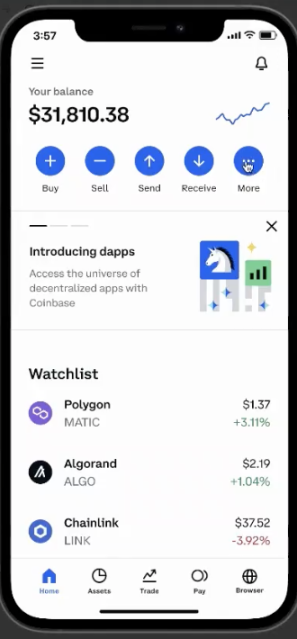This image showcases a cell phone screen displaying a detailed cryptocurrency management interface. The phone's status bar indicates a nearly full battery and an excellent cellular connection with all bars visible. The time is displayed as 3:57, and underneath, three horizontal lines signify more options.

The primary display reveals an account balance of $31,810.38, highlighted prominently below a series of data points resembling a stock market graph. Four blue buttons are lined up beneath this balance, labeled as "Buy," "Sell," "Send," "Receive," and "More" (represented by three dots).

A highlighted section under the header "Introducing DAPPS" (Decentralized Applications) provides a key feature of the app, encouraging users to explore the decentralized app ecosystem through Coinbase. Above this header, there are three horizontal bars representing different categories. The first bar is filled and contains an icon inside a block depicting a horse, adjacent to three vertical bars within another block. Above this, a yellow star is displayed, while three blue stars and gray bars rest below it. An "X" icon is placed to the right, possibly for closing the section.

At the bottom of the screen is the "Watch List," detailing currencies such as Polygon, Algorand, and Chainlink, each accompanied by their current price. Indicators in green show currencies that have increased in value, whereas red indicates a decrease. Finally, primary icons for phone functions line the very bottom of the screen.